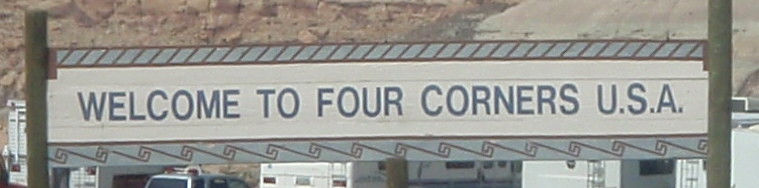The photograph captures a close-up view of a sign that reads "WELCOME TO FOUR CORNERS USA" in bold, all-caps typography. The text appears in a large, bluish-gray font against an off-white background. The top section of the sign features diagonal striping, while the bottom border is adorned with a swirly pattern, adding decorative elements to the otherwise plain sign. The sign is mounted on two poles, positioned on either side—one on the left and one on the right. In the blurred background, a parking lot is faintly visible, dotted with cars and RVs, indicating a busy or well-visited area.